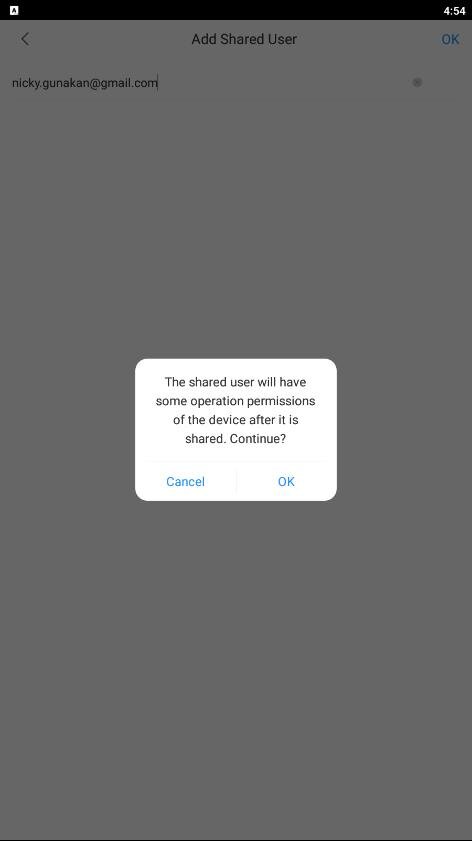The image appears to be a screenshot from a mobile device, likely a phone or a tablet, as suggested by the aspect ratio and the presence of a black status bar at the top displaying the time. The main content of the screenshot shows a pop-up notification overlaid on an application screen.

In the background, the application screen's title at the top reads "Add Shared User" in black text, centered on a white background. Below this title, there is a single input field containing the email address "nikki.gonnacan@gmail.com", entered presumably by the user who initiated the sharing process. The rest of the screen below the input field is largely empty white space, suggesting this part of the interface is waiting for further user interaction.

In the foreground, the pop-up notification is displayed with a semi-transparent gray overlay that slightly darkens the background. In the center of the screen, a light gray dialog box with rounded corners encloses the notification text. The notification informs the user that "the shared user will have some operation permissions of the device after it is shared." The bottom of the dialog box presents two interactive options: "Cancel" and "OK", both rendered in blue text, inviting the user to either confirm or cancel the action.

The status bar at the top left also includes an 'A' icon, which may indicate that the screen is part of an application's settings menu or another administrative interface.

Overall, the image captures a straightforward setup for adding a shared user to a device, with a clear visual focus on obtaining user confirmation through the pop-up dialog.